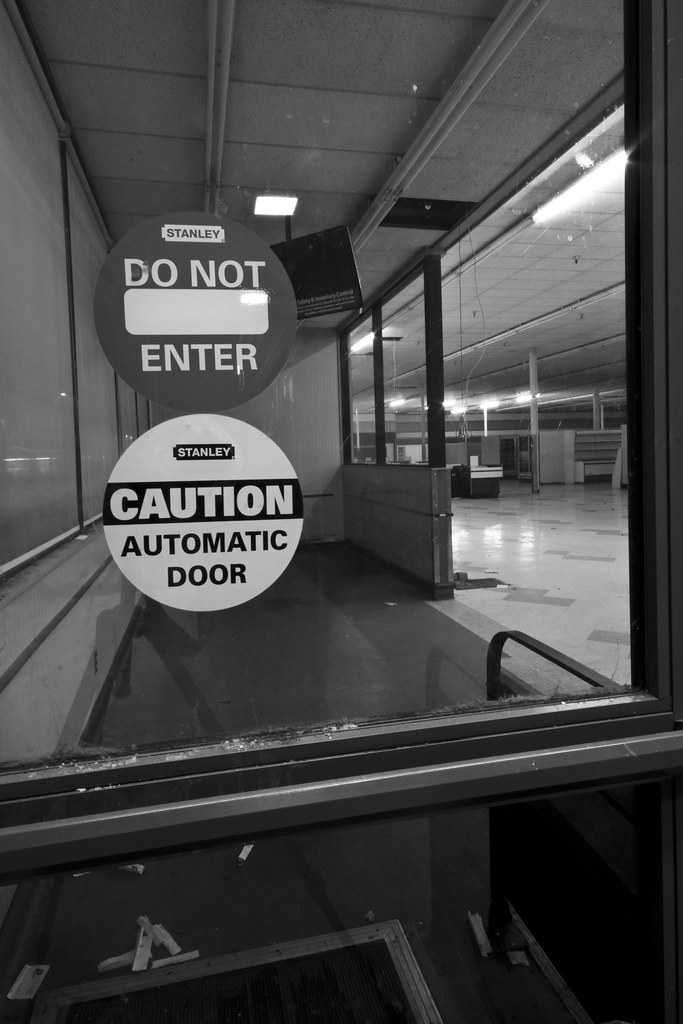This black-and-white photograph features an automatic glass door with a dark frame, prominently displaying two vertically stacked stickers on the middle left-hand side. The top sticker reads "Stanley, Do Not Enter," while the bottom one reads "Stanley, Caution, Automatic Door." The door occupies approximately the top two-thirds of the image, with a divider at the bottom that resembles the solid base of a window. Surrounding the door, you can observe part of a station interior, including white floor tiles, white ceiling lights, and metal guardrails. In the background, past the glass door, there are elements associated with a subway or train station, such as a waiting area with benches and a monitor likely used for tracking departures and arrivals.